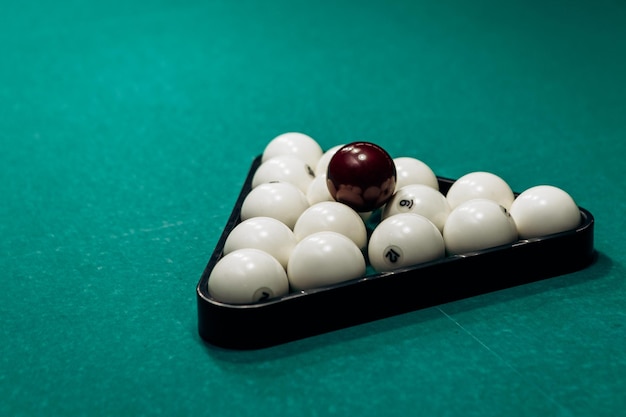This image depicts a set of billiard balls arranged on a teal-colored pool table. The balls are positioned in a black triangular frame with the apex pointing slightly to the top left of the image. Most of the balls are white, each featuring black numbers encircled in the middle, with visible numbers including 12 and 9. Notably, a dark red, almost maroon ball rests atop the white balls. The table surface, extending beyond the mid-ground and foreground, lacks visible boundaries, pockets, or walls, but includes some white lines and light reflections. The grouping of 15 balls appears set up for an initial break shot in a game of billiards.